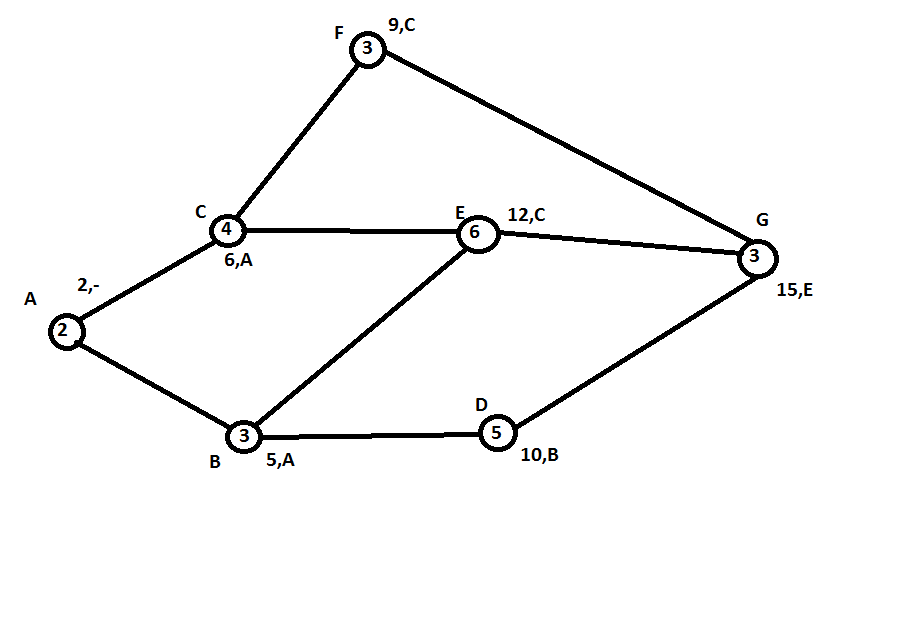The diagram illustrates a network graph consisting of seven interconnected nodes labeled A through G. Each node is depicted as a small circle containing a specific number, and each node also has an additional number outside the circle. Here is a detailed breakdown of the node connections:

- Node A, marked with the number 2 inside the circle, has connections to:
  - Node C, which contains the number 4 inside the circle.
  - Node B, which contains the number 3 inside the circle.
- Node B, in turn, connects to:
  - Node E, which contains the number 6 inside the circle.
- The network ultimately terminates at Node G, which contains the number 3 inside the circle.

Straight lines represent the connections between these nodes, forming a detailed network graph showcasing how each node interrelates and the specific values contained within and outside each node.